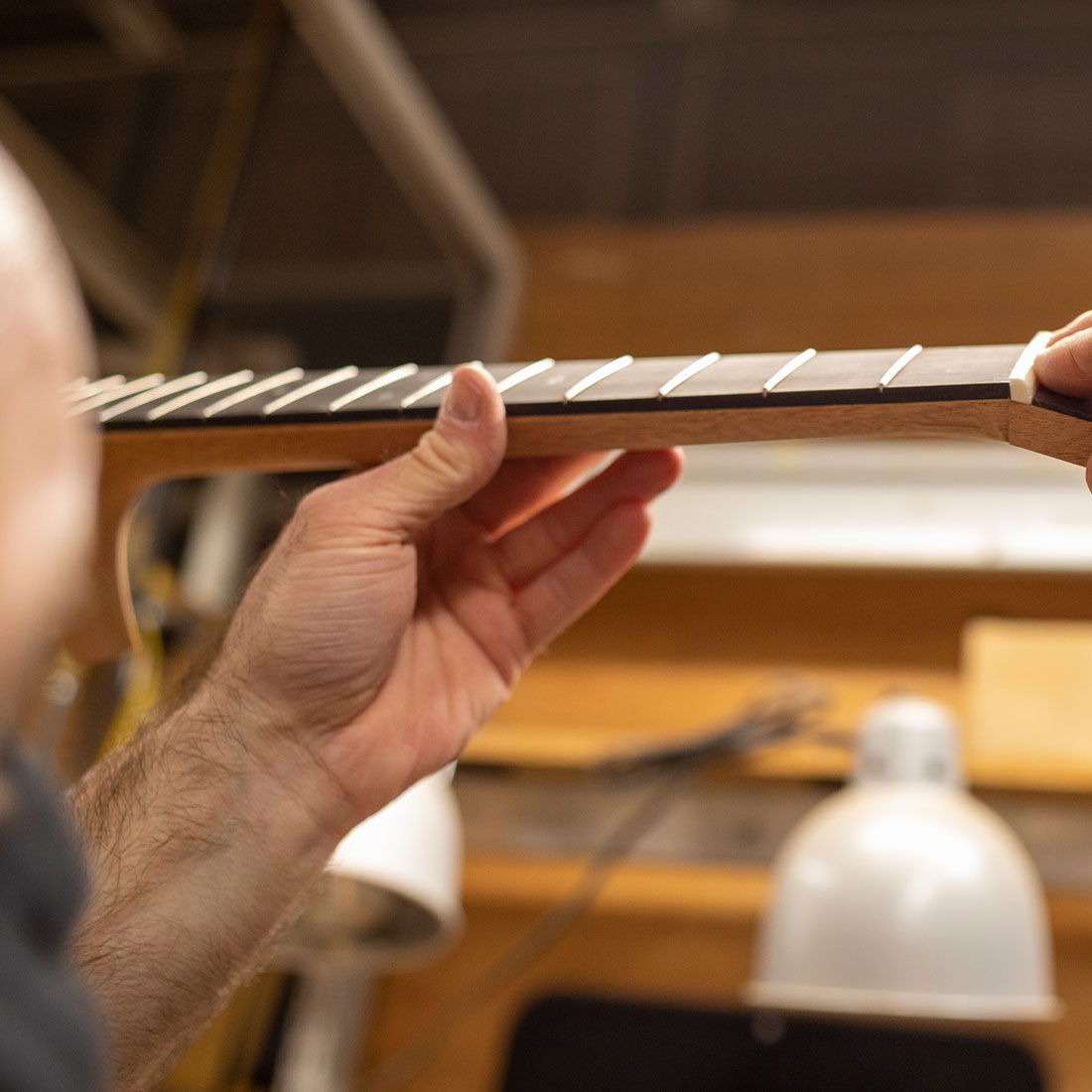In the detailed photograph, a stringed instrument technician, likely male based on the visible hand and partial bald head, is carefully truing the neck of an instrument. The instrument, which could be a guitar or possibly a bass guitar given its narrow shape, is depicted without any strings, revealing only the medium brown wood and the silver frets crossing its neck. The technician's left hand, noted for being somewhat hairy, supports the neck while his other hand holds the headstock. The background is blurred, but a white aluminum desk lamp is visible towards the bottom right. Surrounding the lamp are wooden materials, hinting at the ambiance of a woodshop. The technician appears to be wearing a blue shirt, fitting the workshop environment. The image captures the meticulous craft of instrument building amidst a workspace filled with intriguing, albeit blurred, details.